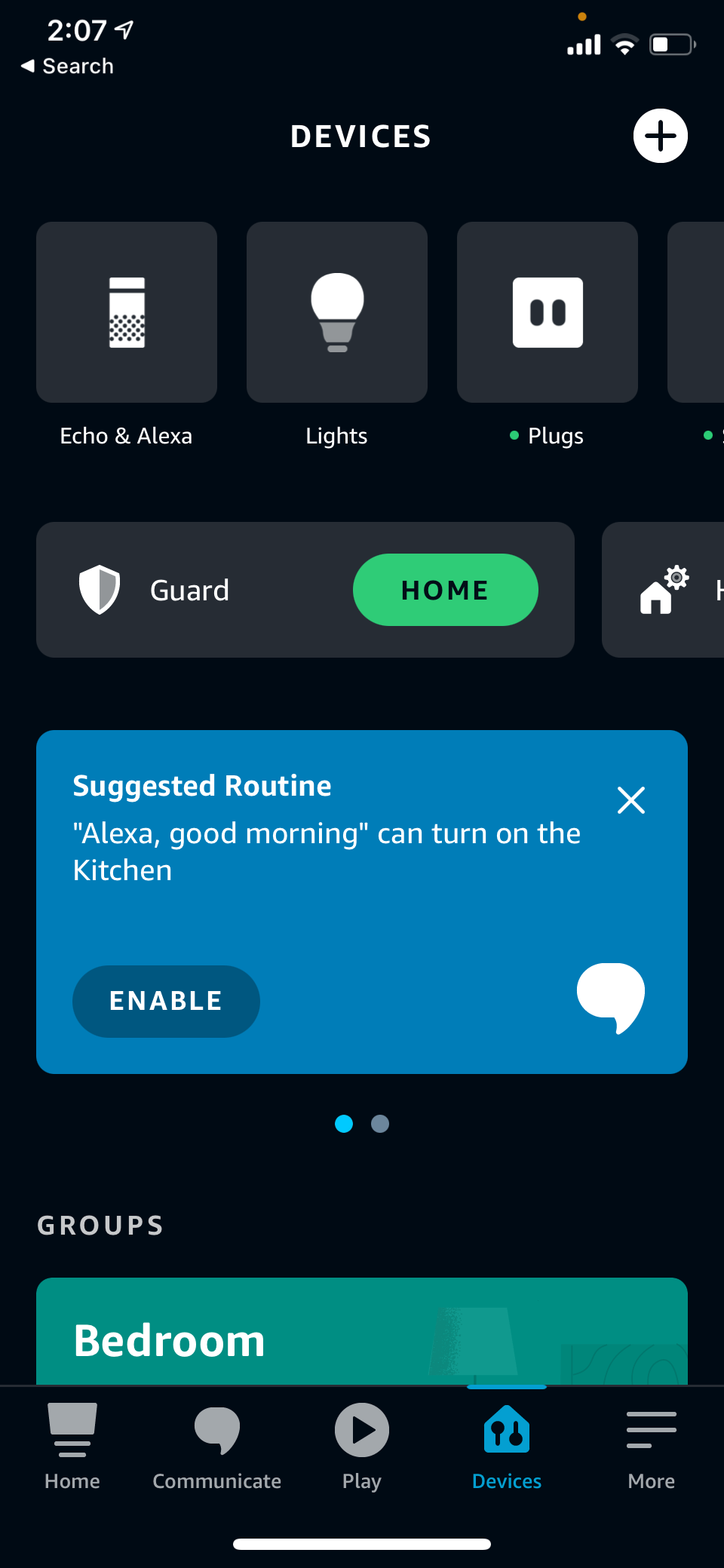This image is a screenshot from a mobile device, specifically showcasing the "Devices" page of a smart home application.

At the top center, the word "Devices" is prominently displayed in white font. To the right of this text, there is a white circle containing a black plus sign. Below this header, there are three horizontally aligned sections or "blocks" labeled "Echo & Alexa," "Lights," and "Plugs," which represent different categories of connected devices.

Underneath these blocks, an additional section labeled "Guard" appears. Adjacent to this is a green button labeled "Home." To the right, partially cut off by the edge of the image, is another block that includes a home icon and a gear icon, indicative of further settings or options.

Further down the screen, there is a blue box highlighting a 'Suggested Routine.' This routine is titled "Alexa, good morning" and is designed to turn on the kitchen lights. An "Enable" button is also present within this blue box, inviting the user to activate this routine.